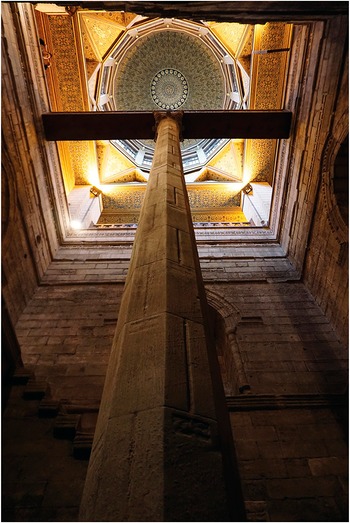The interior photograph captures the awe-inspiring architectural splendor of what appears to be a Romanesque or Gothic era building, possibly a church. The camera is angled upwards towards the center of a vibrant, intricately designed dome that showcases an array of colors, including white, yellow, greens, and ornate patterns. The dome, ornate with floral designs and intricate patterns, stands resplendent under modern lighting which illuminates its colors vividly. At the center of the photo, a massive stone column, which might also incorporate some wood, rises up to support the structure. Surrounding this central feature, the interior side walls are constructed from a mix of gray stone and red and white brick, which ascend to soaring heights of around 80 feet. The space below is a tight, square area, emphasizing the verticality and grandeur of the structure. The combined elements suggest a fusion of Romanesque and Gothic architectural styles, with an air of historical significance and meticulous craftsmanship.